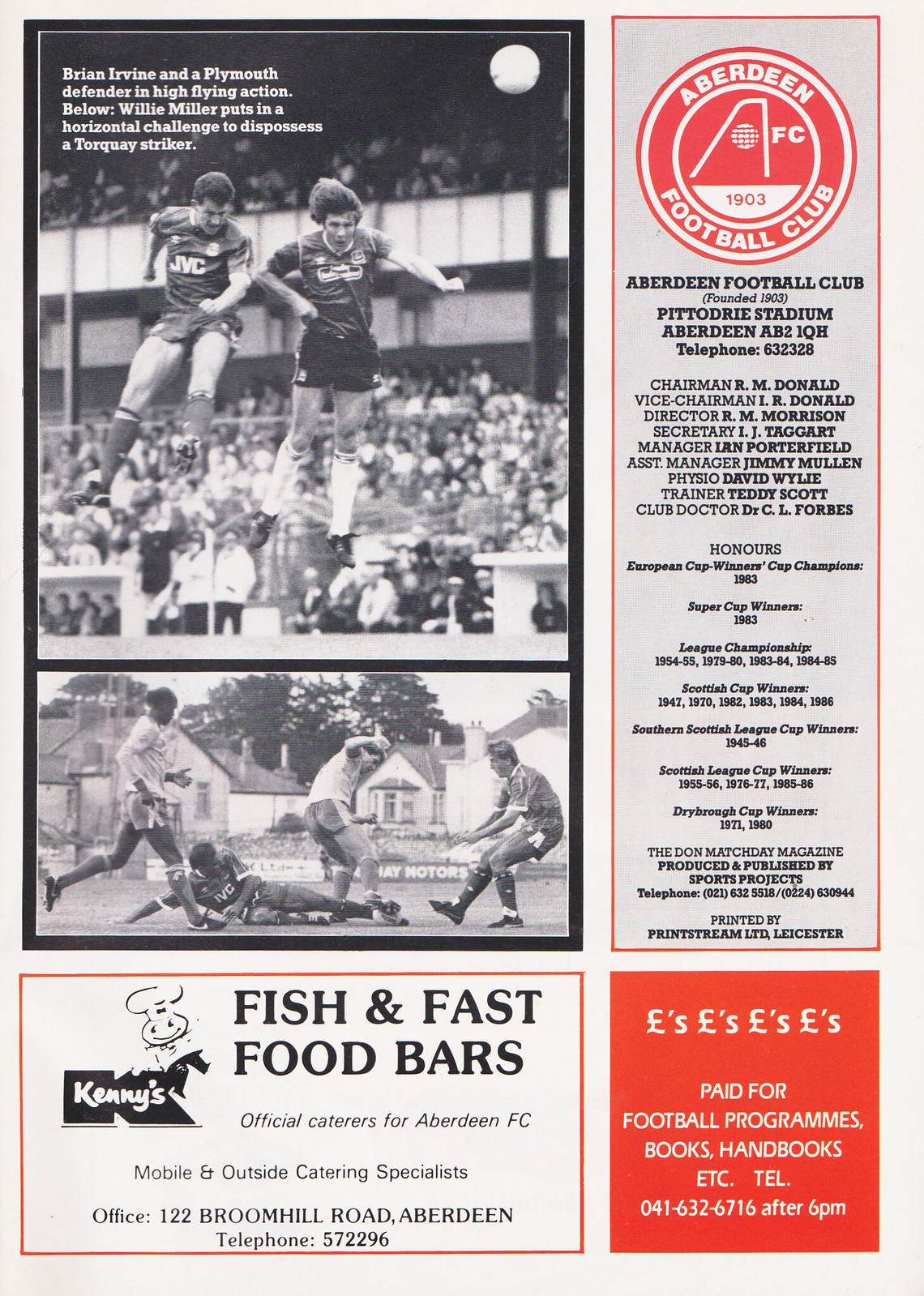This vertical rectangular image, resembling a page from a magazine or pamphlet, prominently features content related to Aberdeen Football Club. At the top left, a black and white photograph captures two soaring soccer players with a white ball in motion, set against the backdrop of a packed stadium. Below this, another black and white image depicts soccer players, one of whom is on the ground, with houses visible in the background instead of an audience. Small printed text within the images reads, "Brian Irvine and a Plymouth defender in high flying action" and "Willie Miller puts a horizontal challenge to dispossess a Torquay striker." Below these photos is an advertisement for Kenny's Fish and Fast Food Bars.

On the right side, the Aberdeen Football Club's round, white and red logo is positioned at the top. Beneath the logo, extensive print details various members of the organization, stating: "Aberdeen Football Club, founded 1903, Pittodrie Stadium, Aberdeen AB2 1QH, telephone 632-328. Chairman RM Donald, vice chairman IR Donald, director RM Morrison, secretary IJ Taggart, manager Ian Porterfield, assistant manager Jimmy Mullen, physio David Wiley, trainer Teddy Scott, club doctor Dr. C.L. Forbes." An additional advertisement in red is located in the lower right corner.